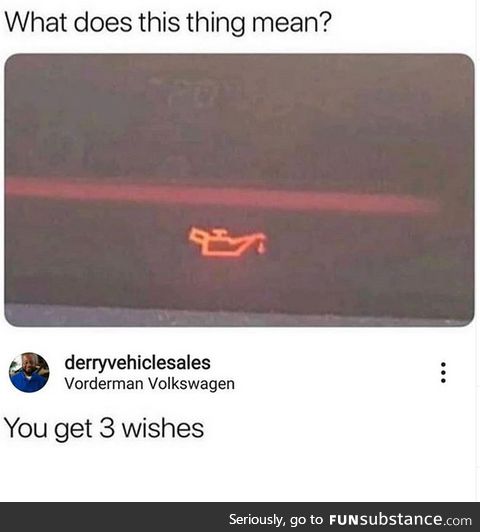The image appears to be a meme originating from a specific website, with a humorous overlay and descriptive elements. At the top of the image, in black text against a white background, is the question: "What does this thing mean?" followed by a question mark. Directly below this text, there is a zoomed-in photograph of a car dashboard displaying an illuminated oil indicator light, which resembles a genie's lamp with a drop of oil dripping from it. This orange icon stands out against the dark dashboard.

Beneath the photograph, a social media reply is included. The responder’s handle is "Dairy Vehicle Sales, Vorderman Volkswagen," and the profile picture depicts a smiling black man wearing a blue collared shirt. The reply humorously states, "You get three wishes." 

Finally, at the bottom of the image, a black bar runs horizontally with white text that reads, "Seriously, go to funsubstance.com." This message is repeated for emphasis.

The overall composition of the image is designed to deliver a humorous take on the car’s oil indicator, drawing a parallel to a genie's lamp granting wishes, and promoting the website funsubstance.com.